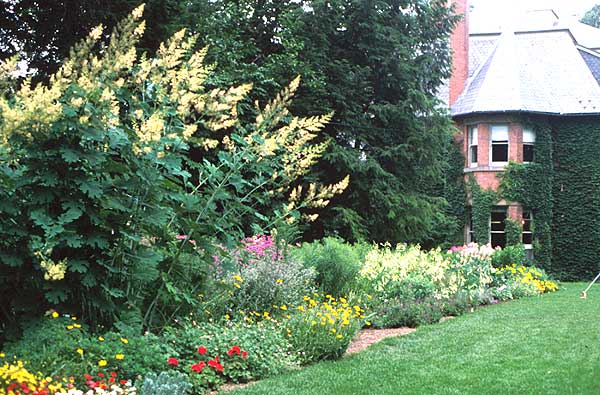This photograph captures a beautifully maintained backyard garden adjacent to an old-style two-story brick house. The house features a distinctive turret with six windows—three on the upper floor and three on the lower—partially covered with lush green ivy and dark green moss. A chimney extends from the side of this turret, adding to the historic charm of the building, which boasts a light gray, shingled roof.

In the foreground lies a meticulously mowed lawn, transitioning into a mulched garden area. This garden area is populated with a vibrant array of flowers and plants. In the lower sections, a variety of colorful flowers are visible, including yellow daisies, red and pink roses, and perhaps some white and purple blooms, all creating a lively border. 

Towards the middle and back of the garden, taller green plants with yellow-tipped leaves rise above the lower flowers. Standing at the rear, there are larger green trees, possibly pine, enhancing the garden's lush scenery.

Adding a further touch of enchantment to the scene is a hint of a pink house with a white roof visible in the background, partially obscured by the garden's verdant growth. This charming, vibrant garden and historic house make for a picturesque and serene outdoor setting.